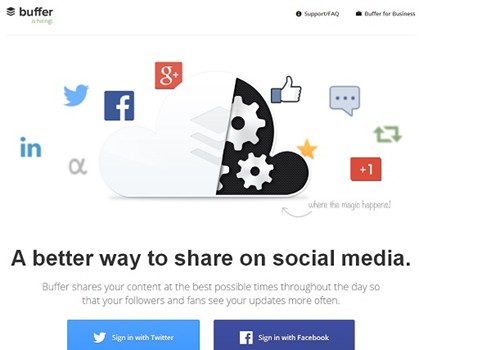The image appears to be an advertisement for Buffer, a social media management tool, designed to be shared on social media platforms. At the top left of the image, the brand name "Buffer" is prominently displayed. On the right-hand side of this section, there are two black text options: "Support FAQ" on the left and "Buffer for Business" on the right.

Below this, icons for various social media platforms including Twitter, Facebook, Google, and LinkedIn are displayed, indicating possible integrations or sharing options.

The right-hand side of the image features a black background adorned with various icons. These include two silver, gear-like wheels, a thumbs-up symbol, a message icon, a Google+ "plus one" symbol, a red square, a yellow star, and two revolving arrows in gray, suggesting interaction and engagement.

At the bottom of the image, a tagline reads "A better way to share on social media." Underneath this, in very small gray text, it states, "Buffer shares your content at the best possible times throughout the day so that your followers and fans see your updates more often," highlighting Buffer's key feature of optimal content scheduling.

Two call-to-action buttons are positioned at the bottom left corner. The left button, in light blue, says "Sign in with Twitter," while the right button, in dark blue, says "Sign in with Facebook." The remainder of the image has a clean white background, providing a clear contrast and emphasizing the central content.